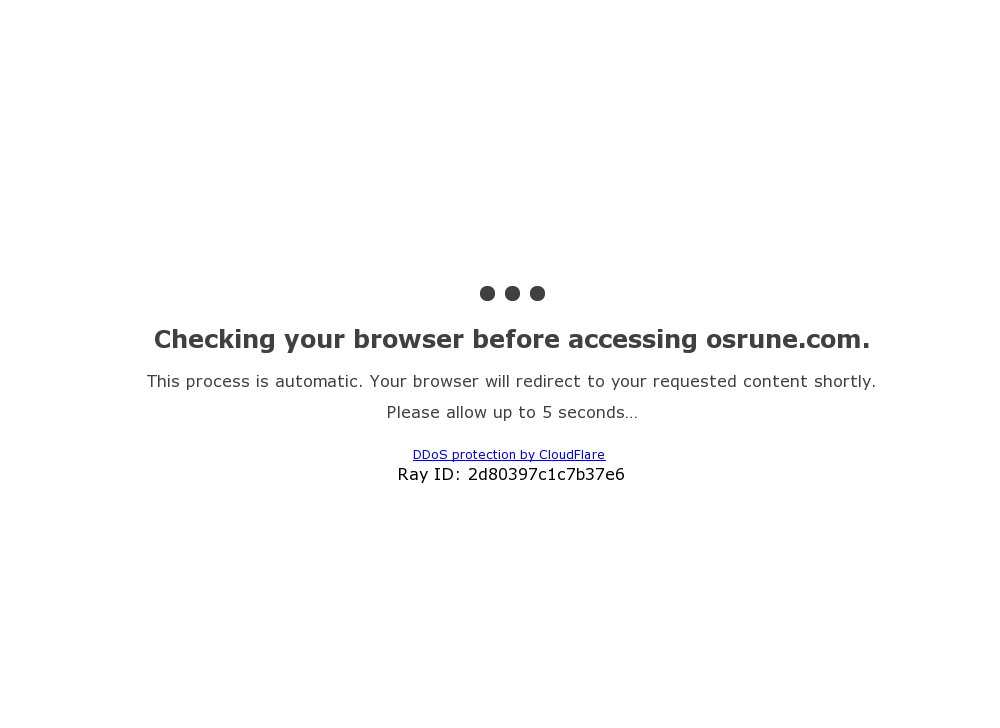The image displays a pre-website loading screen designed to verify system functionality before allowing access to osrune.com. Positioned at the top center are three horizontal dots. Below this, in bold black text, it reads "Checking your browser before accessing osrune.com." Following this primary message, a smaller black font states, "This process is automatic. Your browser will redirect to your requested content shortly. Please allow up to five seconds..." There is an underlined link in blue text that reads "DDoS protection by Cloudflare," signifying the employing of security mechanisms. At the bottom of the image, in small black text, is the identification code "Ray ID: 2d80397c1c7b37e6." The entire image features a stark white background with no borders, and the only element in color is the blue Cloudflare link, making it stand out against the monochrome text.